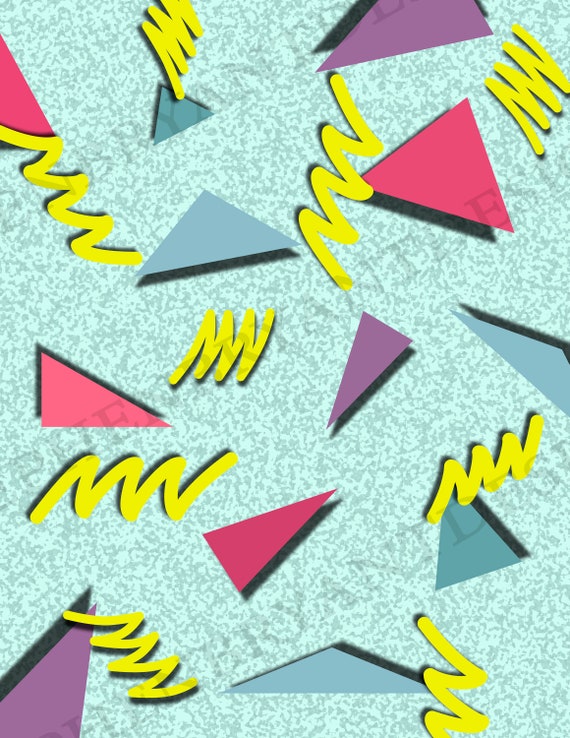The image features a vibrant, 90s-inspired design reminiscent of the style seen in the TV show "Saved by the Bell." The background is a seafoam green with darker green speckles, creating a textured look. Scattered across this background are various geometric shapes, predominantly triangles in shades of blue-green, pink, and purple. Each triangle has a subtle black shadow, giving them a three-dimensional effect. Among the triangles, there are yellow squiggly lines resembling lightning bolts, adding a dynamic feel to the composition. The layout is portrait-oriented, and there's a faint, diagonal watermark across the image, with some letters, like the letter 'E', partially visible over the solid-colored triangles. There are no people or text in the image, just the playful arrangement of geometric patterns and bright colors, capturing an unmistakable 80s and 90s aesthetic.